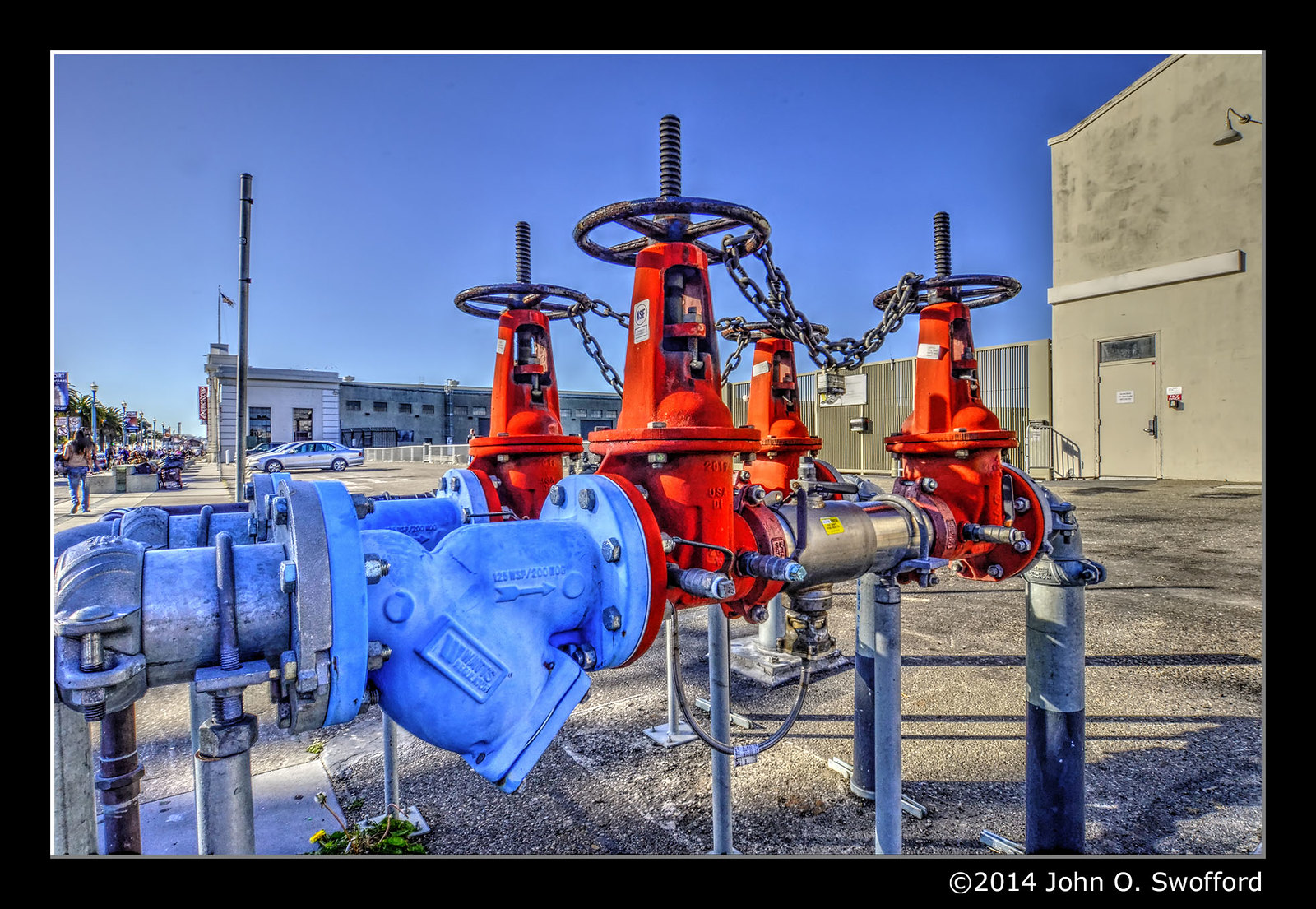The image displays an outdoor scene dominated by a complex network of industrial pipes and valves situated in what appears to be a concrete or asphalt parking area. In the foreground, there are two sets of interconnected pipes, each set featuring two large red valves with chained turn wheels to prevent unauthorized use. The pipes, primarily painted a faded light blue, extend from the ground, connect, and then re-enter the ground. One of the blue pipes includes a blue connecting union to the left of the second red valve. The entire piping structure is supported by steel poles. Rivets securing the connections are visible, contributing to the industrial feel of the setup.

In the background, a gray concrete building rises to the top of the image on the right side, while additional one- and two-story buildings, some displaying flags, can be seen to the left. The area appears to be part of a busy urban setting, with people walking around and cars parked alongside the buildings. Additionally, a single door and a work light are visible on one of the structures. The sky is depicted as clear with a nice blue hue. The photograph is framed by a black border, and the bottom-left corner contains the copyright notice "© 2014 John O. Swofford."